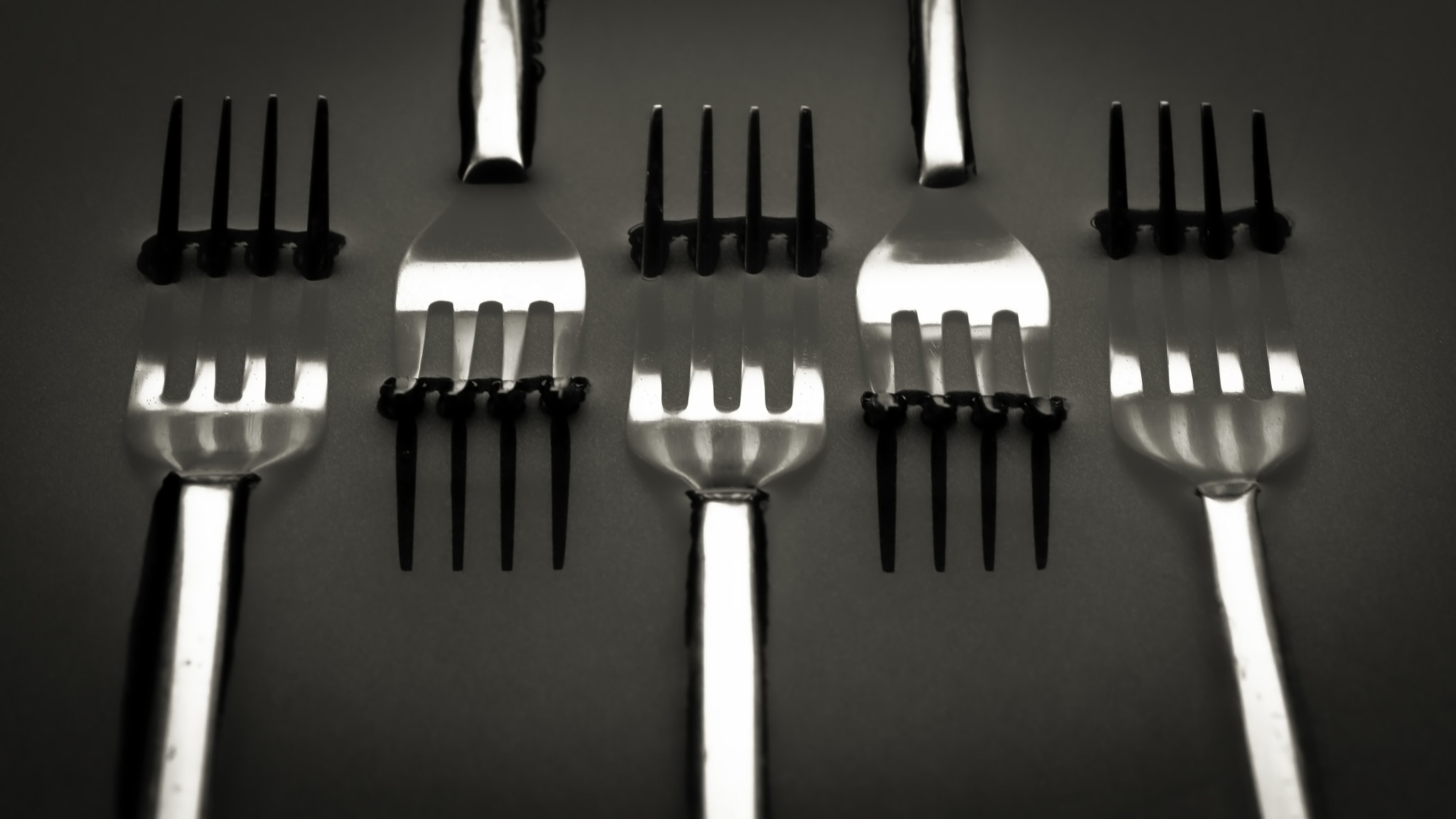This image depicts an artistic arrangement of five silver-metallic forks set against a dark grey backdrop. The forks, appearing new with cardboard weaved through their tines, are positioned in an alternating orientation: the handles and tines face different directions in a sequential manner. Starting from the left, the first fork's handle points down while its tines are upright. The next fork is oriented in the opposite direction, with the handle up and the tines pointing down, continuing this alternating pattern. Reflective highlights are evident on the handles and just below the tines, adding brightness to the otherwise dark composition. The forks are designed with a mix of silver metal and black accents, further accentuating their intricate arrangement. The dark grey background subtly lightens near the forks, creating a visual gradient that emphasizes the forks' artistic and modern presentation.